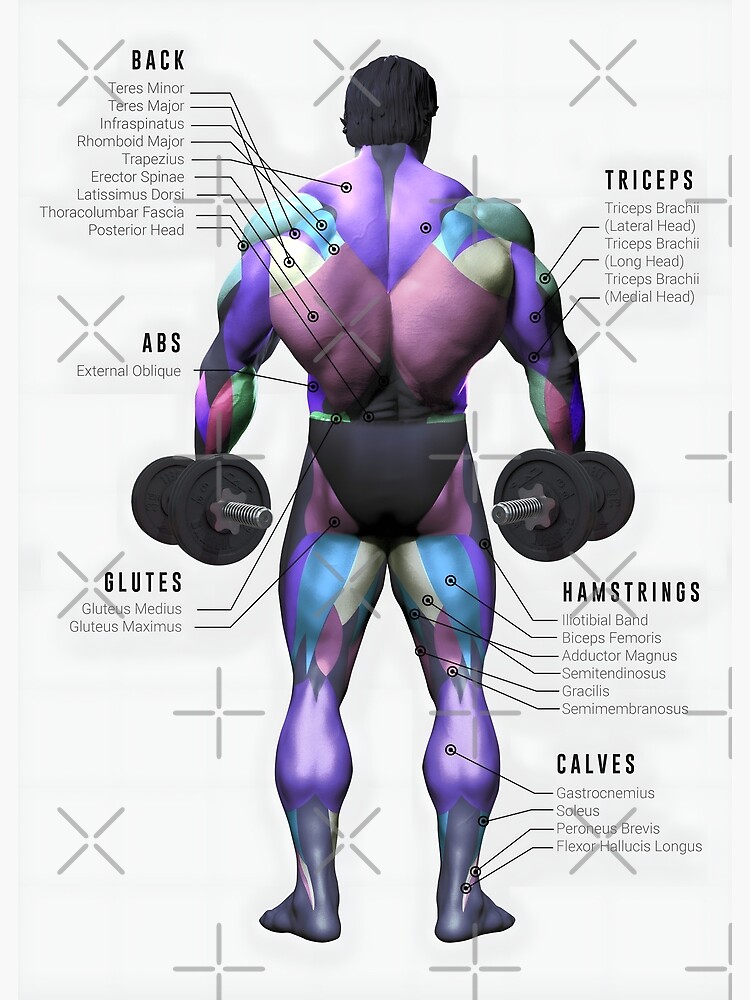The image displays a detailed poster of a very muscular man with his back turned. The man's body, depicted in striking shades of purple, pink, and blue, is intricately labeled to highlight various muscle groups. Each muscle group is clearly marked with black labels, featuring headings such as back, abs, glutes, triceps, hamstrings, and calves. Arrows point to the respective muscles, with labels like gluteus medius and gluteus maximus providing further specificity.

The man is holding grey dumbbells in both hands and is dressed in either underwear or a fitness uniform. The background is a subtle greyish-white, setting a tone that aligns with fitness, health, or gym environments. This meticulously labeled diagram serves as an educational tool, spotlighting the complexities of the human muscular system.